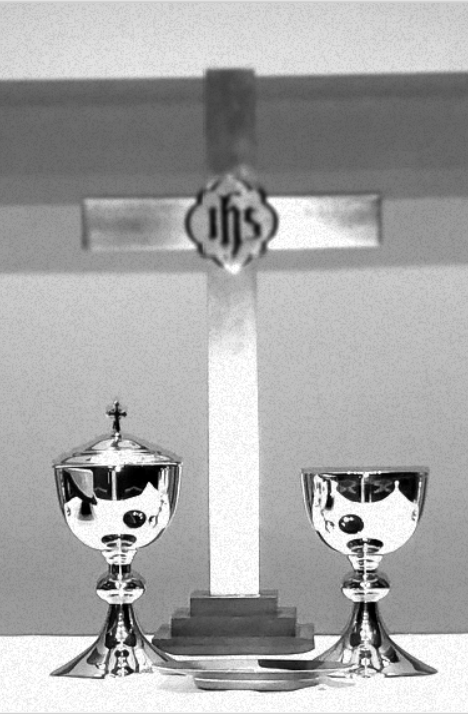This black and white photograph captures a detailed close-up of a religious setting, likely within a church. Centrally positioned is a prominent silver cross on a pedestal, with a rounded plaque at its intersection bearing the letters "IHS". Flanking the cross are two shiny silver chalices; the one on the left has a lid adorned with a tiny cross, while the other is identical but without a lid. Between the chalices sits a small silver plate. The reflective nature of the chalices presents subtle shadows and hints of the surrounding table. The scene is meticulously composed, emphasizing the ceremonial objects against a simple wall background, suggesting a setting for a communion service or similar religious event.